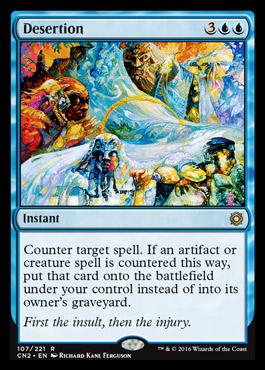This portrait-format, color illustration depicts a detailed card from a role-playing game. The card, titled "Desertion," features an elaborate and mysterious illustration combining elements of snowy mountains and towering giants, rendered in vibrant and intriguing hues. The card includes a message that reads: "Instant – Counter target spell. If an artifact or creature spell is countered this way, put that card onto the battlefield under your control instead of into its owner's graveyard." Below the main text, in italic script, it states: "First the insult, then the injury." The card is copyrighted by Wizards of the Coast in 2016.